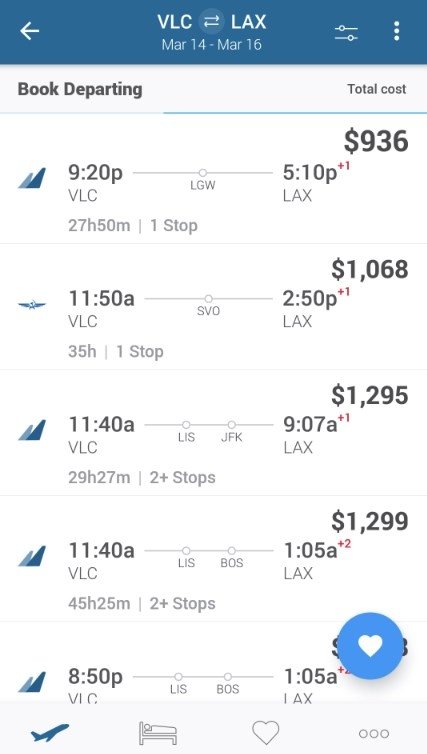An itinerary summary is displayed with a distinctive blue border at the top. Within this border, there is an arrow pointing left and a title that reads "VLC to LAX, March 14th through March 16th." A vertical ellipsis is placed on the right side of this border. The section below transitions into a clean white background where the details of the travel options are laid out in a two-column format.

The left column is titled "Book Departing," while the right column is labeled "Total Cost." Listed in order from top to bottom in the left column are various flight options with specific details:
- The first option shows a departure time of 9:20 PM from VLC, a travel duration of 27 hours and 50 minutes with one stop, arriving at 5:10 PM in LAX.
- The next option lists a departure from VLC at 11:50 AM, a total travel time of 35 hours with one stop, to LAX.
- Another option departs from VLC at 11:40 AM, taking 29 hours and 27 minutes with two or more stops, arriving at LAX.
- The last option depicts a departure at 8:50 PM from VLC, arriving at LAX at 1:05 AM after a yet-to-be-specified duration.

In the right column, the corresponding prices for these flights are presented:
- The first flight option is priced at $936.
- The second option costs $1068.
- The third option is available for $1295.
- The final option lists a price of $1299.

This detailed itinerary provides a comprehensive overview for travelers planning their journey from VLC to LAX between March 14th and March 16th.